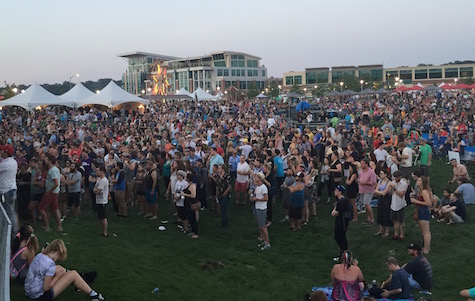The image depicts a large outdoor event, possibly a concert or festival, taking place on a grassy field during what appears to be the late evening of a summer day. The crowd, comprising hundreds or possibly thousands of people, is mostly standing and facing towards a presumed stage situated off to the left side of the image. A few individuals are seated on the grass, some looking at their phones. The attendees are dressed in light, muted summer clothing such as shorts and t-shirts, suggesting it is warm. The overall color scheme of the image is muted with no overly bright colors. Multiple tents—white, red, and gray—are scattered around the field, indicating areas likely designated for food or other services. In the background, a substantial building resembling a university campus or similar large facility is visible. The sky is overcast, adding a slightly dim ambiance to the scene.